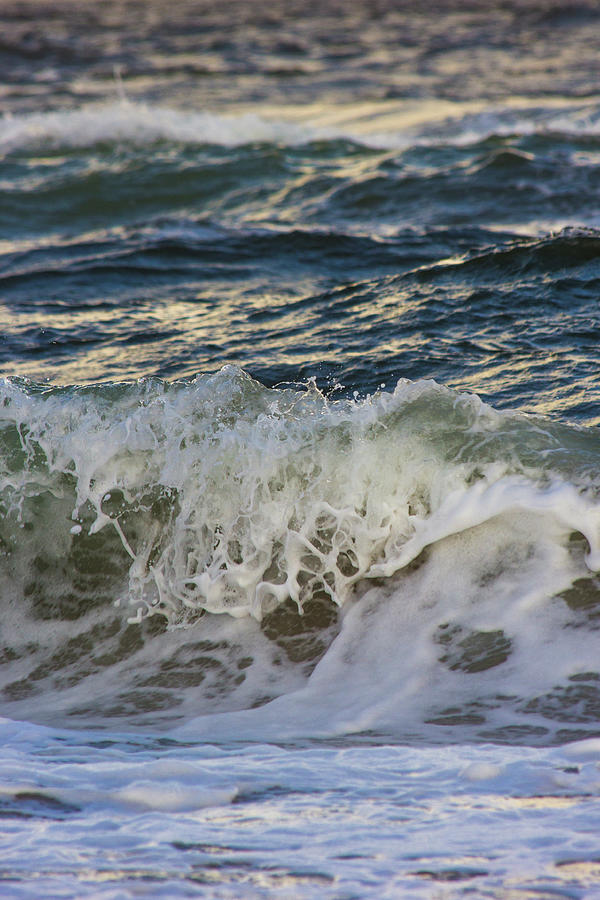This image captures a close-up of an ocean wave dramatically crashing, with a strong emphasis on the frothy whitewater that characterizes the scene. The wave, about two feet tall, is in sharp focus, highlighting its curling tip and the churning foam created by its breaking action. The surface of the water is turbulent, covered with white foam, indicating either windy conditions or the aftermath of a recent storm. Further back, the ocean appears slightly out of focus, revealing additional white caps floating on the dark blue water, which reflects a warm, yellowish light suggesting the time of day to be near sunrise or sunset. The entire background of the image transitions into a blur, enhancing the texture and intensity of the foreground wave, while the absence of the sky and beach places sole attention on the tumultuous, sun-kissed, and dynamic water.